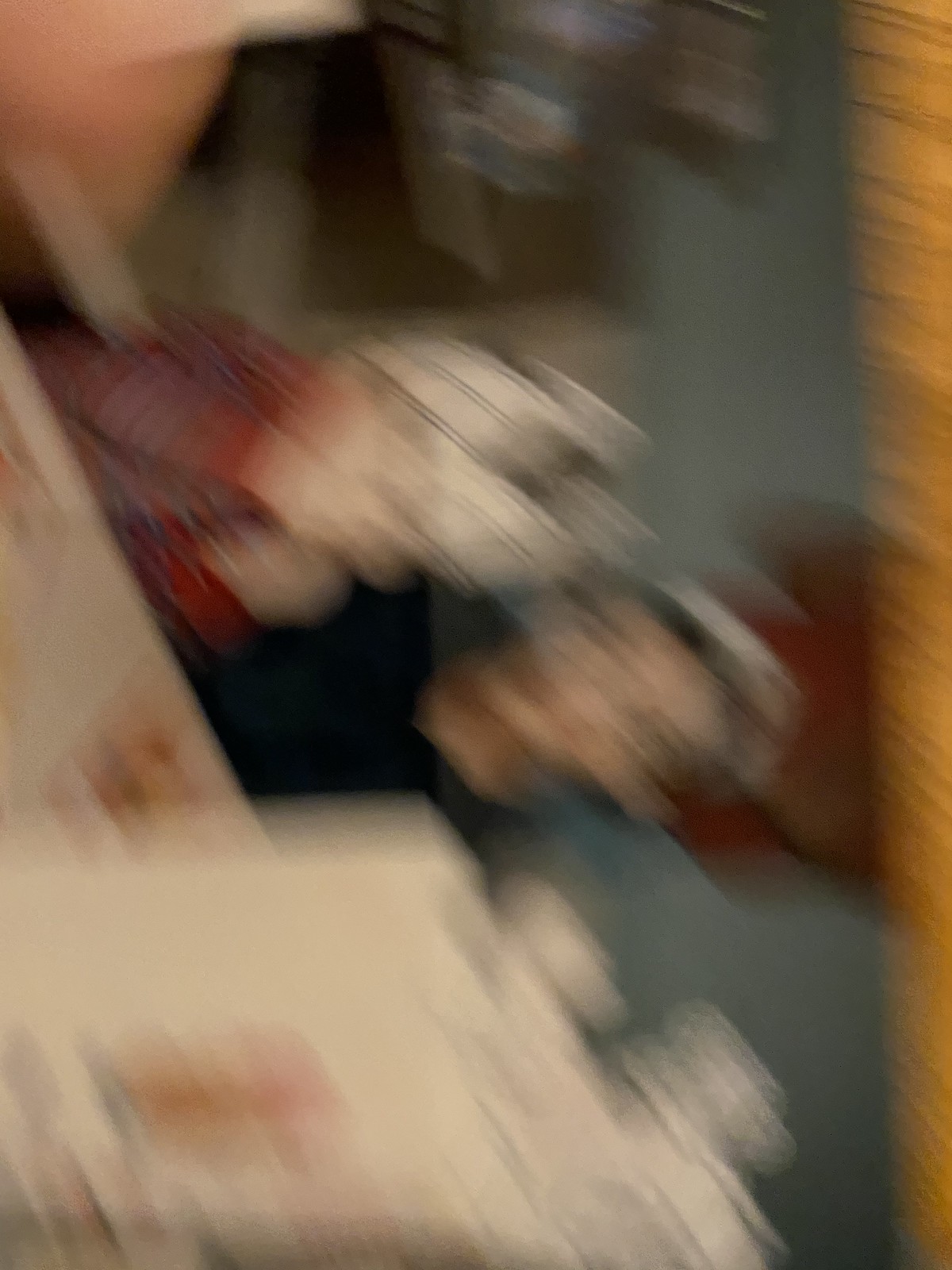A blurry, poorly oriented photograph features two children, one in a black shirt and the other in a red and blue striped shirt, possibly wearing paper hats. To view the image correctly, it should be tilted 90 degrees to the left. In the foreground and to the lower right, there is a white box adorned with red and orange designs. The background is predominantly dark, suggesting the image was taken in a dimly lit room.